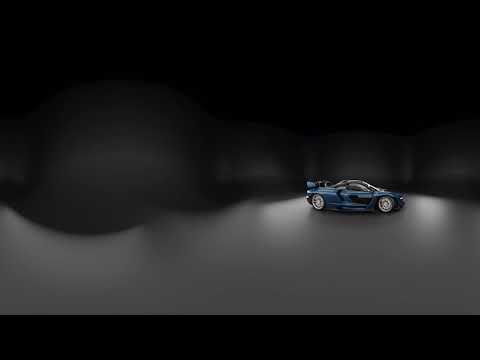The image is a horizontally aligned rectangular photograph, bordered in black at both the top and bottom. The background features a predominantly gray abstract design, resembling a large cloud or a tilted chess piece, larger on the left and narrowing towards the right, with a gradient that goes from brownish-gray to gray-black. Below this, there's a middle gray section that represents a floor-like surface.

Positioned slightly to the right of the center sits a sleek, dark blue sports car. The car faces to the right, equipped with a raised spoiler and chrome wheels. This vehicle, likely a two-seater, is highlighted against the abstract background, standing out as if it’s part of a still image from an advertisement. The overall composition presents a modern and artistic style, devoid of any text, with a focus on the contrast of dark hues of black, gray, and blue.